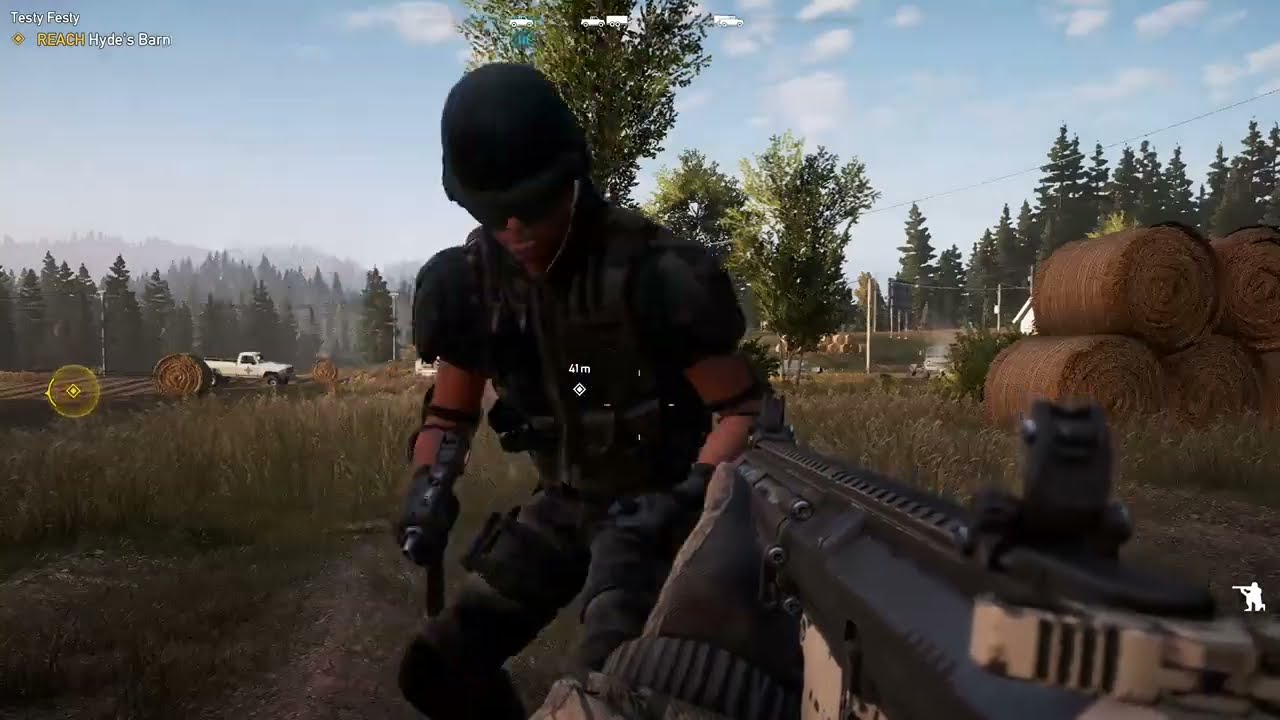The image showcases a scene from a first-person shooter video game set in a sunny outdoor environment with a few clouds in the sky. In the foreground, a player’s gloved hand grips an M16 assault rifle pointed at an approaching enemy character situated roughly 41 meters away, as indicated by an in-game distance marker. The enemy, dressed in black tactical gear and dark glasses, carries an Uzi in his right hand and is advancing toward the player. The background reveals a mix of pine trees, wheat fields, and various bales of hay arranged in stacks, enhancing the rural atmosphere. Additional details include a white pickup truck in the far left background and what appears to be a house and power lines on the right side of the image. The player’s UI features include a compass and a crouching icon, reinforcing the tactical, immersive nature of the game.